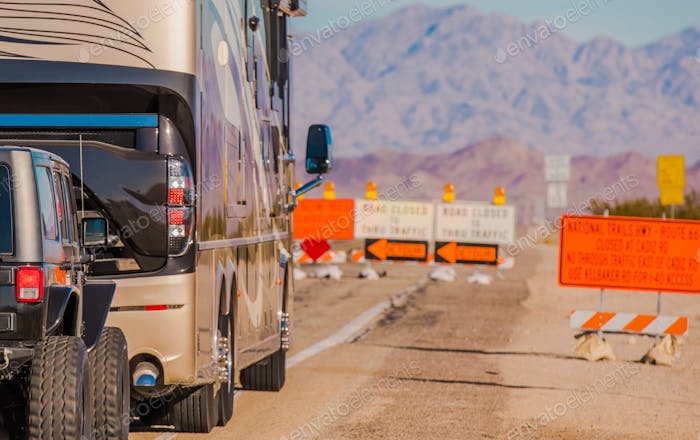The image is a horizontal rectangular photograph depicting a road scene with a clear foreground and a blurred background. On the left side of the image, there is a tan-colored, modern-looking recreational vehicle towing a smaller, black off-road vehicle, likely a dune buggy or a jeep. The road itself appears to be partially paved and tan in color, with a solid white center line. Scattered across the middle of the scene are multiple construction signs indicating the road is closed, with arrows directing traffic to a detour on the left. One prominent sign on the right side is orange with multiple lines of black text that reads, "NATURAL TRAILS ROUTE 66 CLOSED AT," though the rest of the text is blurry. Further back on the right side, there is a large orange barricade. In the distance, sand-covered mountains and sky are visible but heavily blurred, giving a sense of isolation and remoteness. The entire setting suggests a closed road near a mountainous area, with brown, blue, orange, black, white, red, and tan colors dominating the scene.